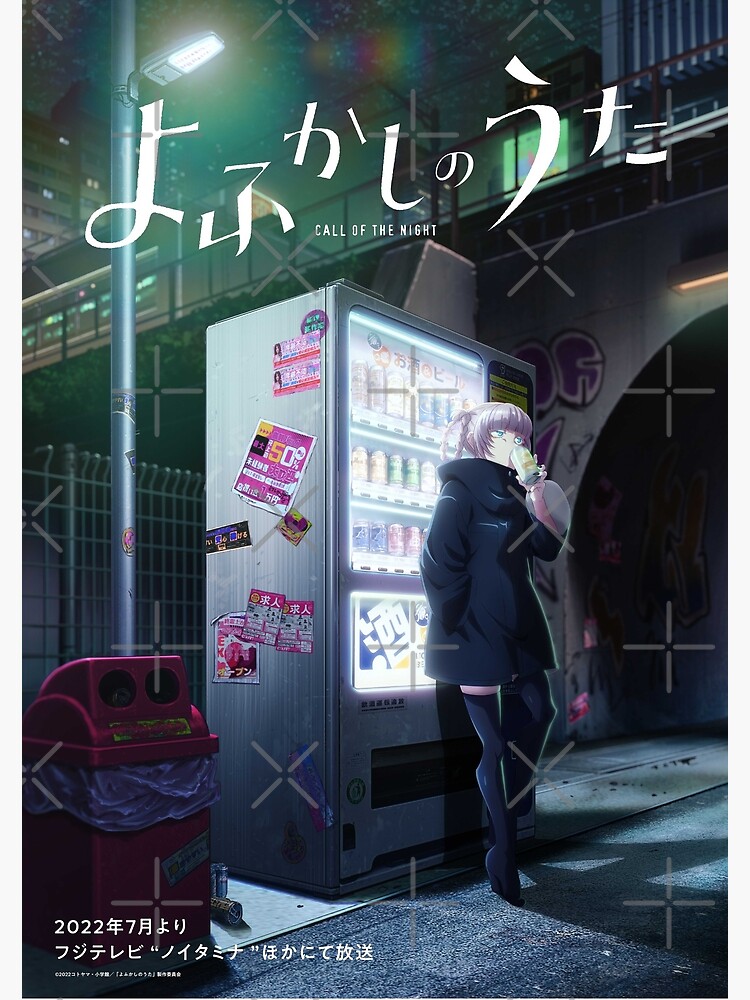The cover illustrates a night scene from the graphic novel or manga titled "Call of the Night," with the title displayed prominently at the top in white Japanese characters followed by its English translation. On the lower left, the date 2022 is visible, along with additional details in Japanese. At the center, a woman is depicted leaning against a vending machine, drinking from a can. She is dressed in a black jacket or hoodie and thigh-high black boots. The setting appears to be an urban nighttime scene, possibly on a sidewalk. Adjacent to her on the left is a vivid red trash can, and a lamppost illuminates her figure and the vending machine, casting shadows on the ground. Further details include colorful advertisements on the side of the vending machine and a tall pole with additional advertisements nearby. In the background, you can discern elements of a cityscape, including what seems to be a tunnel and a bridge, hinting at a train crossing.